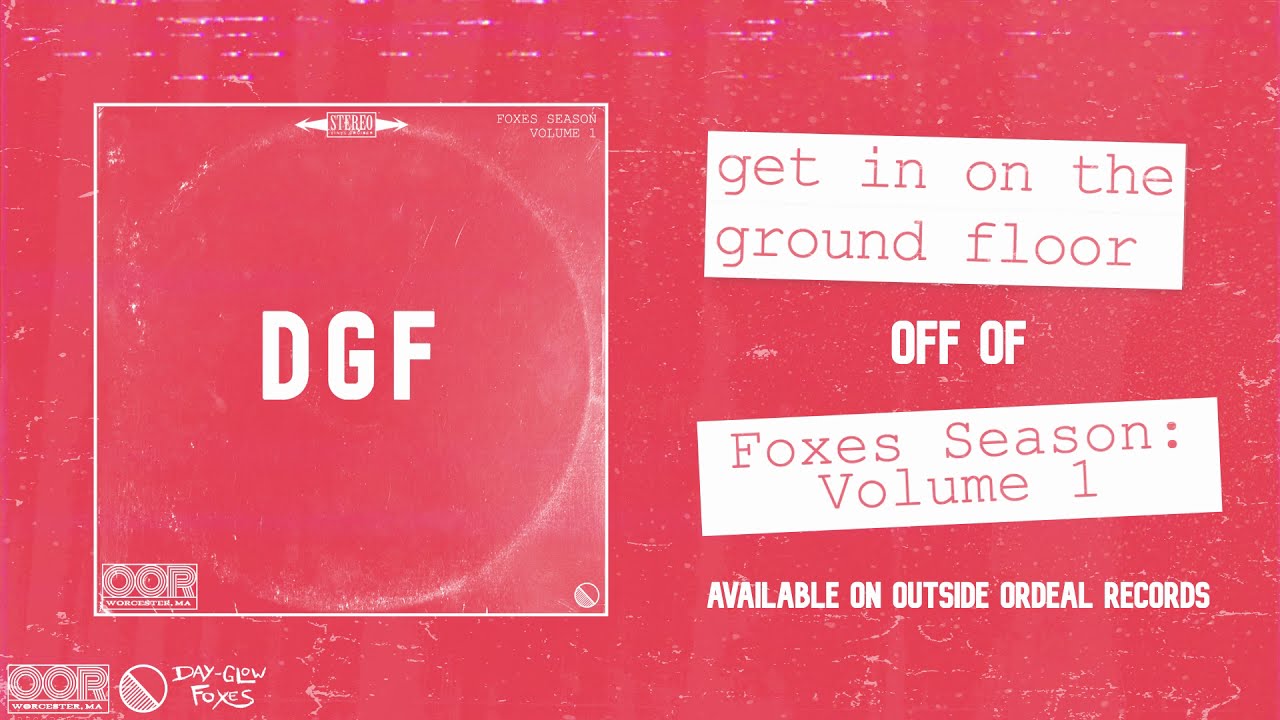The advertisement features a vibrant red background accented with subtle, scattered white lines. Dominating the left-hand side is a square illustration resembling a vinyl record cover, outlined in white with a faint circular design that doesn't quite touch the edges. The center of the square prominently displays the letters "DGF" in large white font, with "Stereo" and arrows at the top, and "Fox's Season: Volume 1" in small text at the upper right corner. The lower section of the square features the logo "OOR." Below this, additional logos display "OOR," a circle design, and the words "Dayglo Foxes" in white font. On the right-hand side of the flyer, the text is presented within white rectangles. "Get In On The Ground Floor" is at the top, followed by "Off Of," "Fox's Season: Volume 1," and "Available on Outside Ordeal Records," all printed in white.